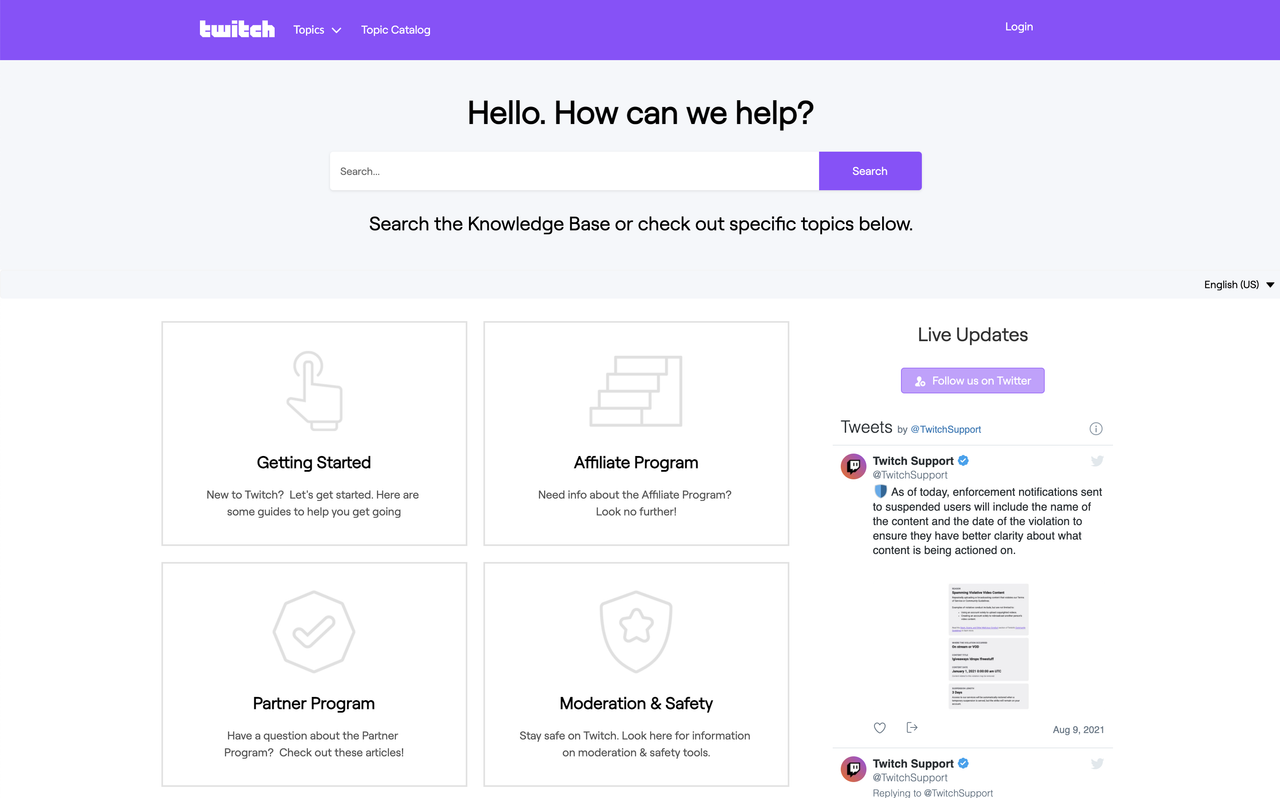The image depicts a webpage, likely from Twitch, a popular streaming platform. At the top left, the Twitch logo is displayed in bold white lowercase "t." On the right, 'Topics' appears in a thinner white font with a drop-down arrow, followed by 'Topic Catalog.' The far-right corner features a 'Login' button.

A light gray bar features a bold black text prompt: "Hello, how can we help?" Below, a URL search bar flanked by a gray 'Search...' placeholder on the left and a purple 'Search' button on the right is visible. Underneath, in bold black text, it reads: "Search the knowledge base or check out specific topics below."

The main section contains four rectangular sections:

1. **Get Started**:
   - Icon: Silhouette of a hand.
   - Bold text: 'Get Started.'
   - Description: "New to Twitch? Let's get started here. Here are some guides to help you get going."
   
2. **Partner Program**:
   - Icon: Hexagonal shape with a check mark.
   - Bold text: 'Partner Program.'
   - Description: "Have a question about the Partner Program? Check out these articles!"

3. **Affiliate Program**:
   - Icon: Staircase.
   - Bold text: 'Affiliate Program.'
   - Description: "Need info about the Affiliate Program? Look no further!"

4. **Moderation and Safety**:
   - Icon: Shield with a star.
   - Bold text: 'Moderation and Safety.'
   - Description: "Stay safe on Twitch. Look here for information on moderation and safety tools."

On the right-hand side is another section labeled 'Live Updates,' with a purple rectangle that includes a silhouette of a person and the text 'Follow us on Twitter' in white. Below, it says 'Tweets' in black, followed by the handle 'By Twitch Support' in blue, alongside the Twitch Support icon featuring a purple and red chat bubble. 'Twitch Support' in bold black with a blue checkmark is displayed next to it.

A gray text bubble indicates: "As of today, enforcement notifications sent to suspended users will include the name of the content and the date of the violation to ensure clarity about what content is being violated." This section includes a small screenshot of a webpage with purple and black text. The first tweet shows a timestamp: "August 9, 2021," at the bottom right corner.